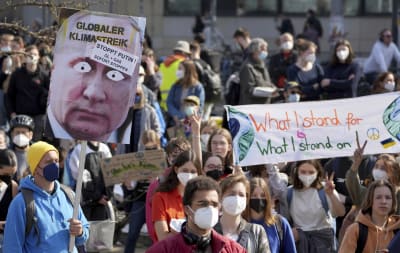The image portrays a peaceful political protest taking place outdoors during the daytime, likely during the COVID-19 era, as almost all participants are donning masks that cover their nose and mouth—predominantly white but also black and blue masks. The gathering consists of numerous individuals marching together, with only a few holding up signs and banners. One prominent placard displays a large photograph of Vladimir Putin with exaggerated googly eyes and text in a foreign language, possibly reading "Globaler Klim Osterreich". Another significant banner reads, "What I stand for, what I stand on". Several demonstrators are seen raising two fingers in a peace sign. In the backdrop, a large, cream-colored building can be vaguely observed, adding context to the scene.